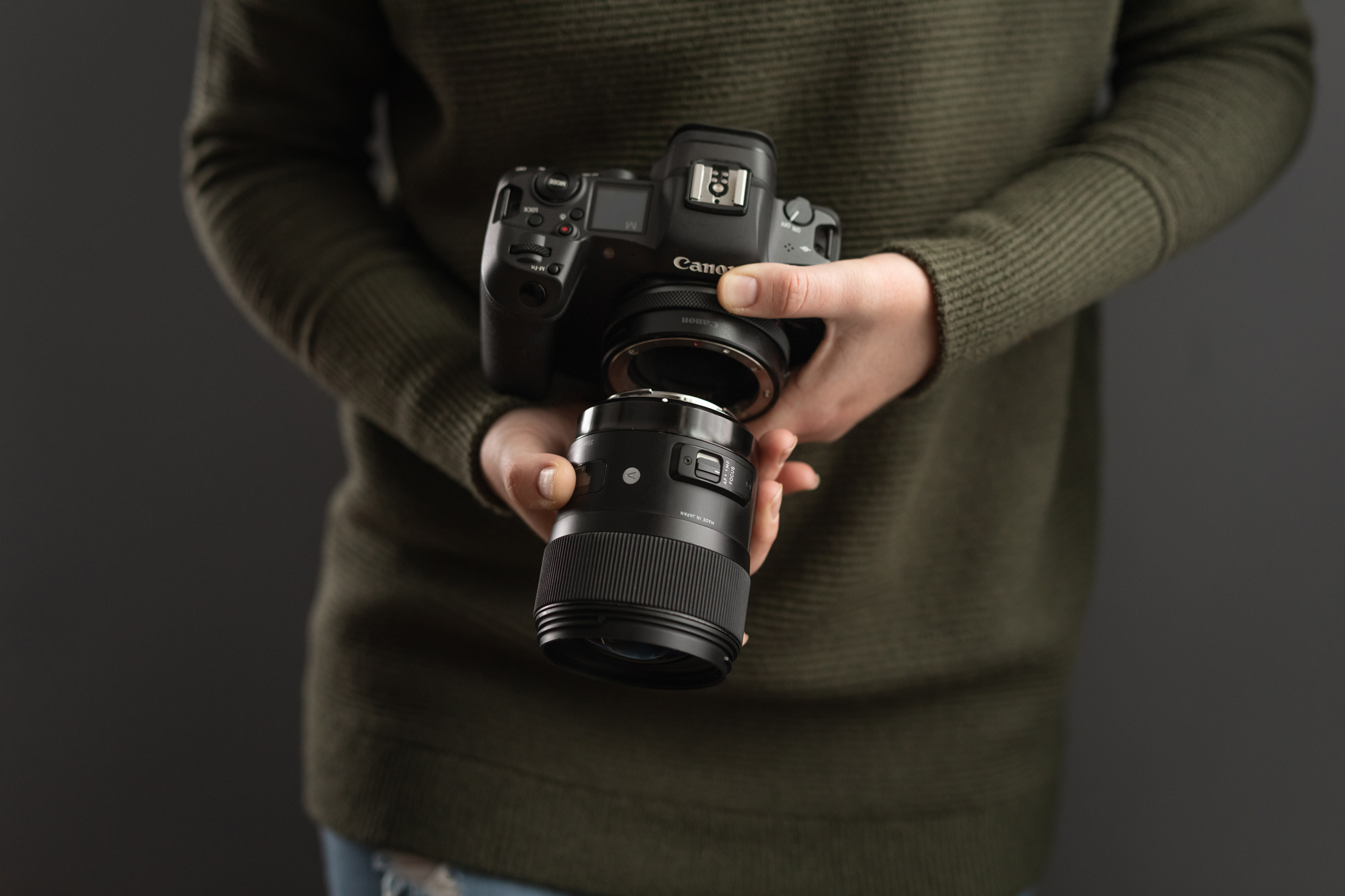In the photograph, there's an individual wearing a green sweater and blue jeans with a visible tear, holding a professional, black Canon DSLR camera. The person's head and neck are out of frame, focusing the viewer's attention on their hands and the camera. Both hands are engaged: the left hand cradles the camera body, while the right hand grasps the lens, which appears to be separate from the camera, indicating that the person might be about to attach it. The individual's thumb partly obscures the Canon logo on the camera body. The lens looks capable of extending further for close-up shots, highlighting the camera's versatility for various photo shoots and situations.